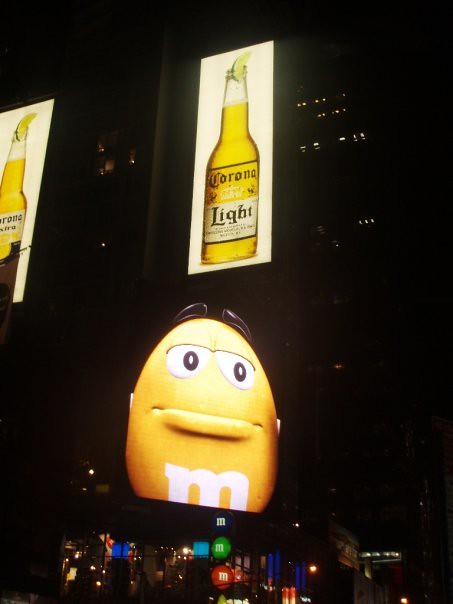The image depicts the yellow M&M's character, known as the Yellow M&M, gazing to the right with black eyes and black eyebrows. Prominently featured on his chest is the iconic white "M" logo. Above him, an illuminated advertisement for Corona Light beer showcases a lime-topped bottle filled with golden beer, accompanied by the Corona Light text. A similar Corona Light advertisement is positioned to the left. Below the Yellow M&M, three other M&M characters—black, green, and red—are displayed. The backdrop presents a nighttime cityscape with office buildings, set in a bustling downtown area, highlighting a large poster of the Yellow M&M character.